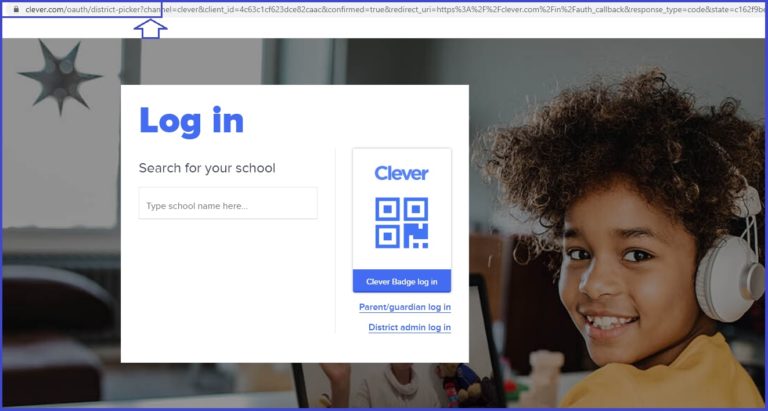A detailed photographic image of a webpage is prominently displayed. At the top, the web address reads "clever.com," indicating it is a secure website, evidenced by the lock icon on the very top left corner. A white pop-up box is superimposed on the page. The header of the box reads "Log In" in a large, bold blue font. Below it, the text prompts users to "Search for your school" with an accompanying input field for users to type in their school name.

To the right of this input field is a slightly smaller square box, which features the word "Clever" written in blue text. This box also contains a QR code and a blue button labeled "Clever Badge Log In." Below this button, there are additional login options labeled "Parent/Guardian Log In" and "District Admin Log In."

Adjacent to the pop-up, a photograph captures a seven or eight-year-old child, smiling brightly over their shoulder. The child, dressed in a blue shirt, has curly brown hair and is wearing white and gray headphones. They are seated in front of a laptop computer, adding a human element to the login page's academic context.